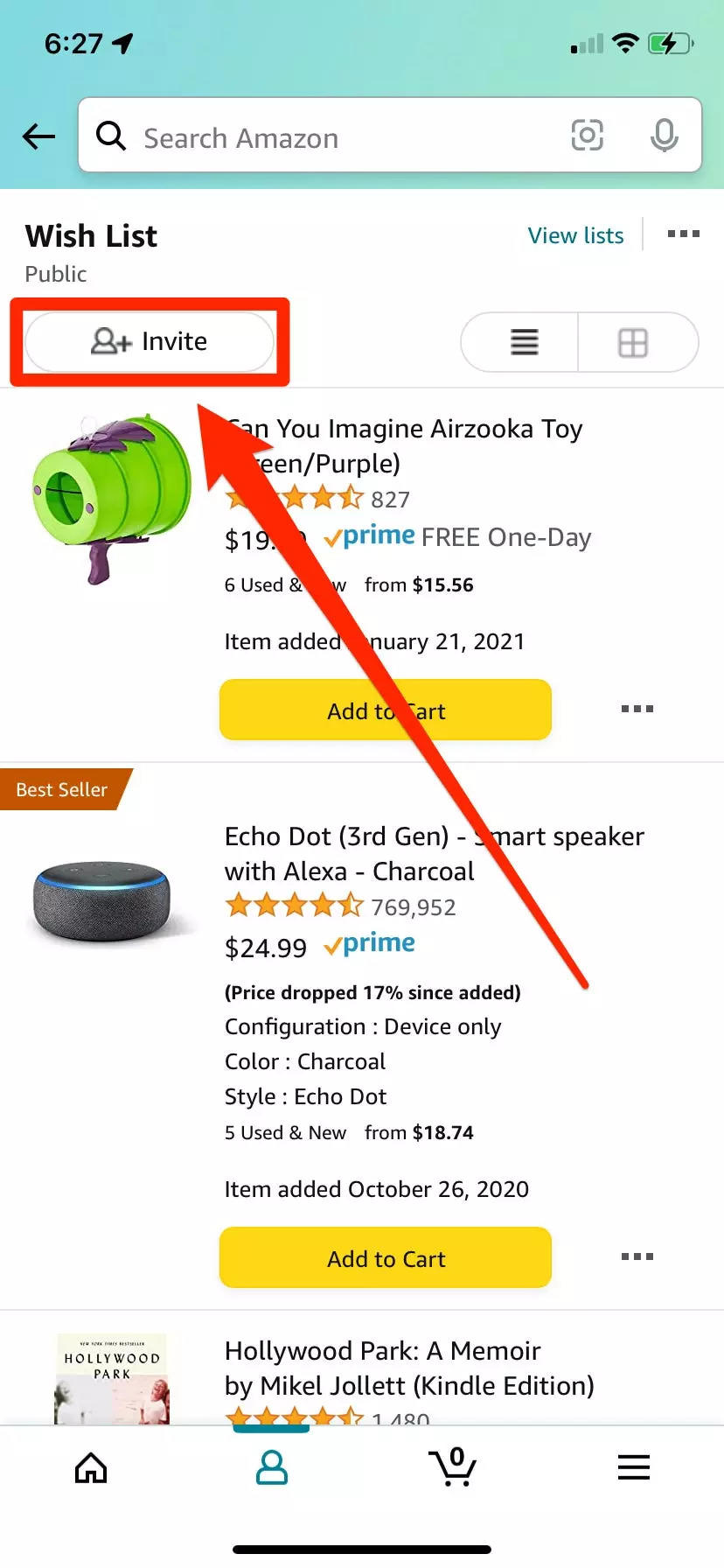The screenshot captured from a mobile device showcases the Amazon app interface, taken at 6:27 AM/PM with location services enabled. The device has minimal carrier signal strength with only one bar, while Wi-Fi is connected, and the battery is approximately 50% charged and currently charging. The screenshot presents the Amazon app's main screen featuring a blue navigation banner at the top.

In detail:
- **Navigation Elements:**
  - *Search Bar*: Labeled "search Amazon" with an accompanying magnifying glass icon.
  - *Icons*: Includes a back arrow, a camera icon for visual search, and a microphone icon for voice search.
  - *Invitation Banner*: An orange arrow labeled "invite," prompting users to invite friends to view a public wish list.

- **Public Wish List Section:**
  - *Header*: "Invite friends to look at your wish list" with a "Visit List" hyperlink in blue font on the right.
  - *Listed Items*:
    1. **Arizuka Toy**:
       - Description: "Can You Imagine Arizuka Toy Green Purple."
       - Visual: A green cone-like toy with a handle.
       - Price: $19.99.
       - Shipping: Free one-day shipping available via Prime.
       - Action: Option to add to cart using a yellow "Add to Cart" button.
    2. **Echo Dot (3rd Generation)**:
       - Price: $24.99.
       - Action: Also available for adding to the cart via a yellow "Add to Cart" button.

This detailed view of the Amazon app highlights the user interface elements, wishlist features, and specific product details, showcasing the app's functionality and user-friendly design.